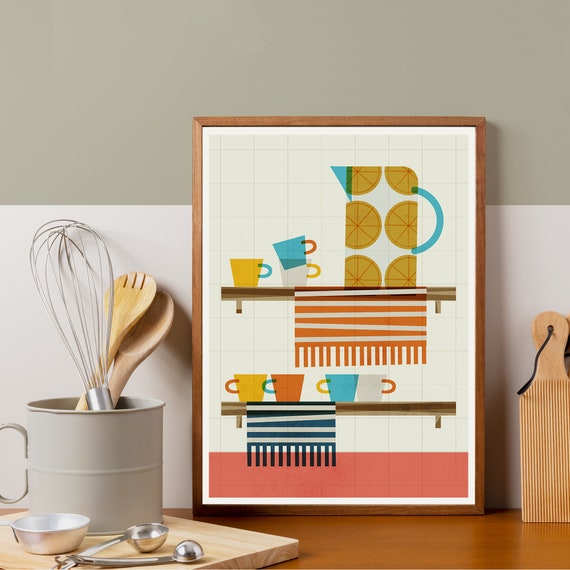This photograph captures a quaint kitchen scene centered around a light brown wooden counter. A picture on the counter features a charming drawing of a lemonade pitcher adorned with illustrations of lemons. To the side, a shelf holds a collection of coffee cups, accompanied by a towel dangling over the edge. Just above, another shelf displays four coffee cups in vibrant hues of yellow, orange, blue, and white, with a blue-striped towel hanging from it. Below, a cutting board is placed next to a tablespoon, teaspoon, and a small bowl. A white tin utensil holder, filled with a whisk and two wooden spoons, adds to the homely feel. Against the white wall, a small wooden cutting board is propped up, completing this detailed and cozy kitchen setup.